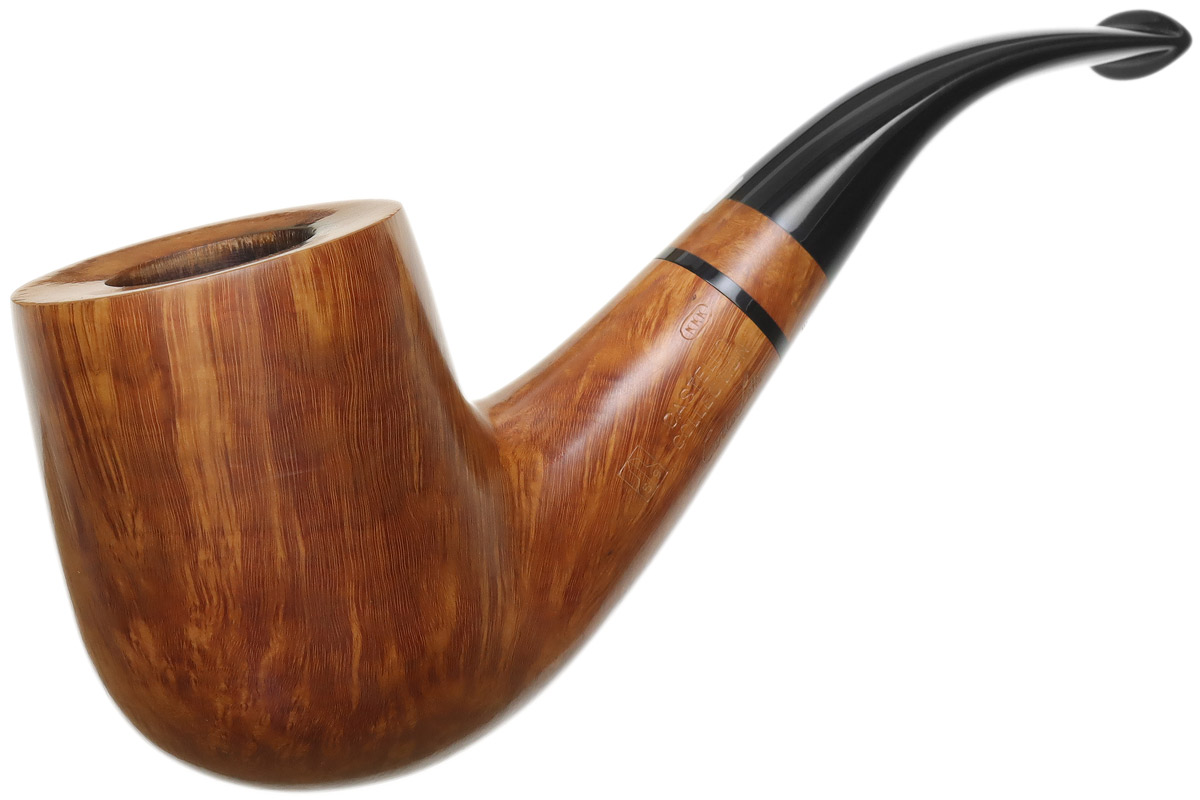This image showcases a traditional wooden tobacco pipe set against a plain white background. The pipe's bowl, where tobacco is placed, is crafted from brown wood with visible wood grains and a lacquered finish, contributing to its smooth, polished appearance. Midway up the pipe's body, a decorative black band encircles it, adding a touch of elegance before the wood continues for a short segment. The pipe's stem, designed for the user to hold in their mouth, is a shiny, solid black material with a slightly tapered end. Notably, the pipe features the letters "KK" engraved on its wooden body, indicating its possible branding or craftsmanship. The overall aesthetic, reminiscent of a style Sherlock Holmes might favor, underscores the timeless appeal of this classic smoking accessory.